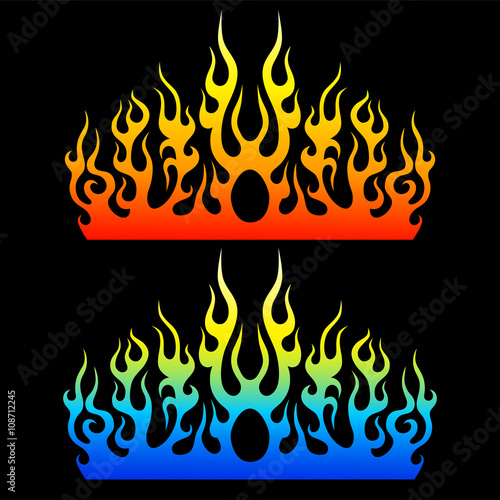Set against a black background, the image features two identical flame-like designs stacked vertically. Both designs resemble stylized crowns with points that resemble flames. The top design starts with a deep orange base that transitions into a gradient of flames, starting from deep orange and fading to yellow at the tips. The bottom design mirrors the top but begins with a blue base, transitioning through lighter shades until it also turns yellow at the tips. Each crown has an egg-shaped hole in the center. Faint gray text reading "Adobe Stock" is scattered subtly across the black background, and vertically along the left-hand side, "Adobe Stock 108712245" is noticeable.